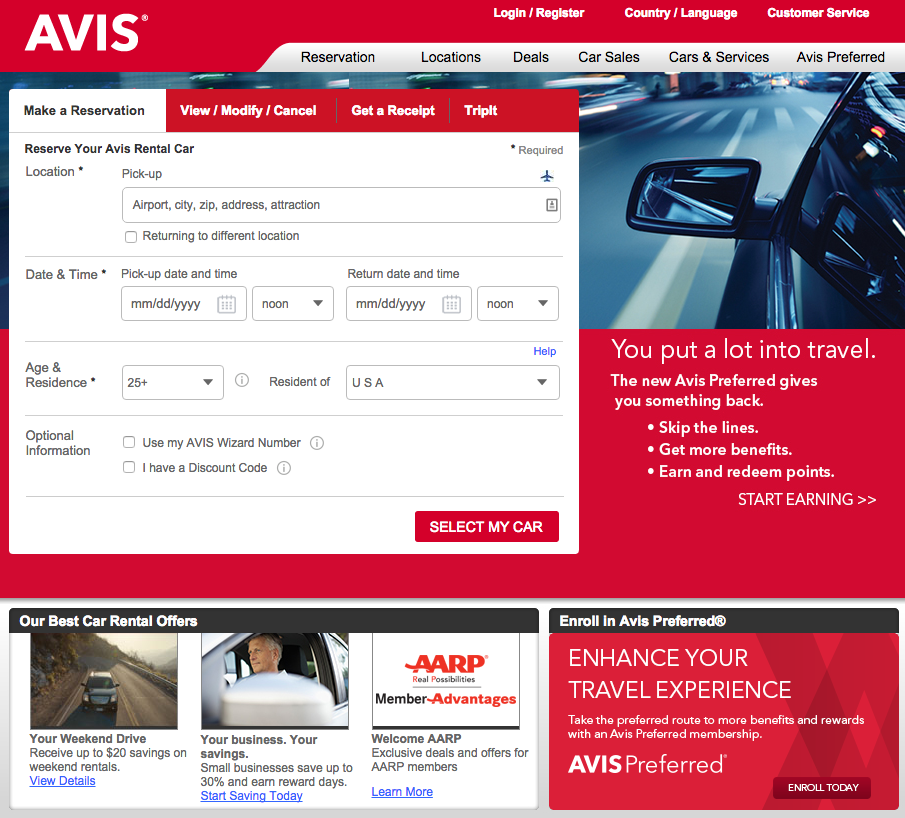Screenshot of the Avis Car Rental website interface, characterized by its distinct red background. The top section prominently displays the Avis brand logo in all capital letters along with navigational links such as "Login/Register," "Country/Language," "Customer Service," "Reservation," "Locations," "Deals," "Car Sales," "Car Services," and "Avis Preferred."

A central white box stands out, featuring the primary function of the site: "Make a Reservation," which is highlighted in white. Additional options within the white box include "View/Modify/Cancel," "Get a Receipt," and "TripIt," displayed with a red highlight. 

The reservation section begins with the prompt "Reserve Your Avis Rental Car" marked with an asterisk indicating required fields. The form includes a location field with a designated box for "Pick Up Location" (also marked with an asterisk). Below the location field, there's an option to "Return to a Different Location," accompanied by a checkbox.

Further down, the form asks for "Pick Up Date and Time," both marked with asterisks, with a date format of MM/DD/YYYY and a dropdown menu preset to "Noon." Similarly, the "Return Date and Time" section follows the same format and options.

Additionally, the form includes fields for "Age and Residence," highlighted with an asterisk. The "25+" age group option is pre-selected, as well as "Resident of USA."

This concise and visually structured interface ensures users can effortlessly navigate and complete their car rental reservations.